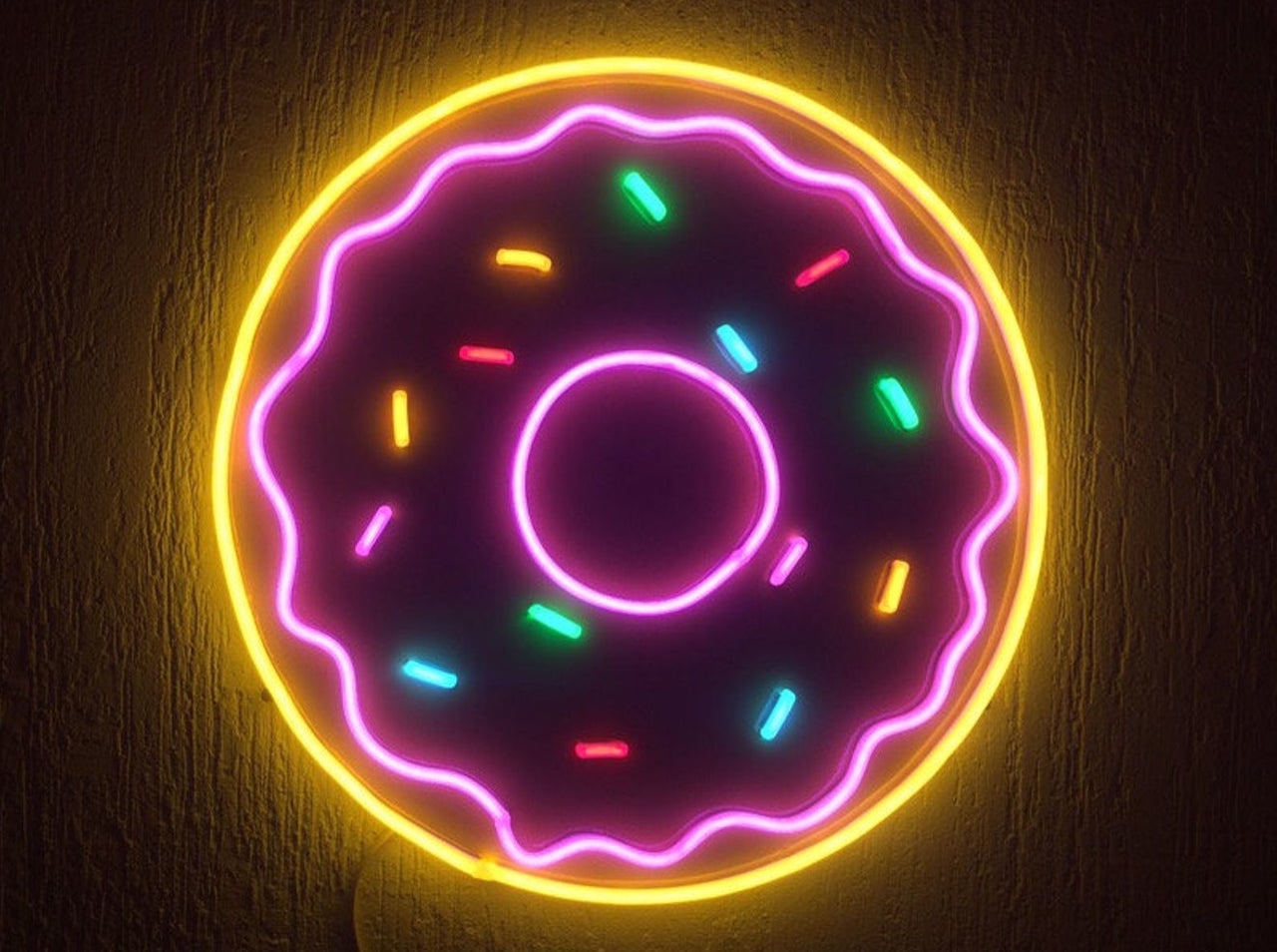This photograph captures a close-up of a vibrant neon sign in the shape of a donut, set against a textured dark brown wood background. The donut design features an outer ring of bright neon yellow and an inner concentric ring of hot pink with a solid pink dot at its center, representing the donut hole. The pink inner line has a swirly, squiggly appearance. Scattered across the donut are neon sprinkles in various colors including green, yellow, red, orange, pink, and light blue. These sprinkles are arranged within the space between the two pink lines. A cord hangs down from the bottom left of the neon sign. The background appears dark, creating a striking contrast with the luminous neon lights, allowing the vivid colors to stand out prominently.